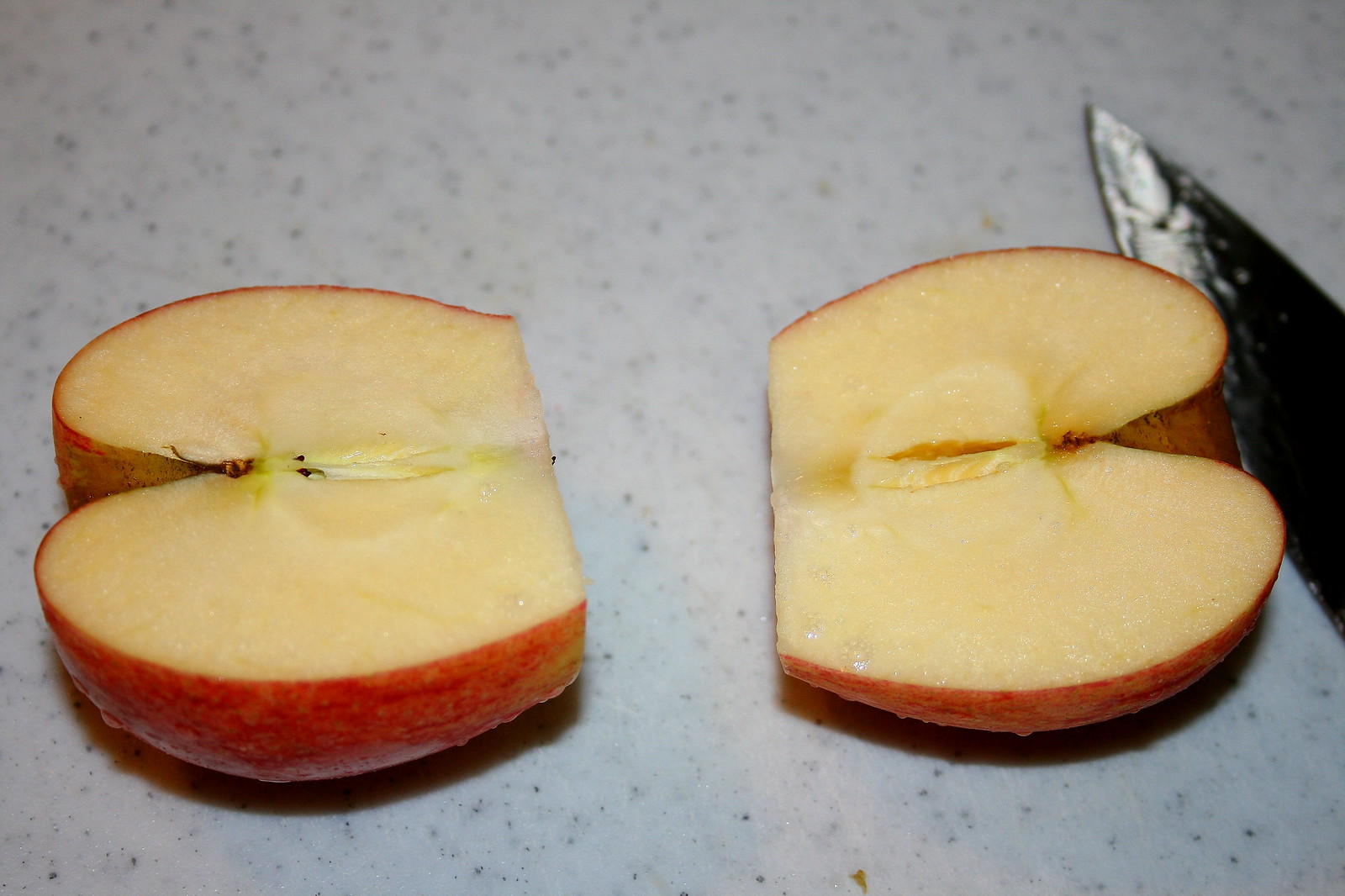A top-down view of a freshly cut apple is presented on a striking marble surface, characterized by its white background peppered with black specks. The apple has been halved and further sliced at the base, creating two pieces that together resemble an abstract heart shape. The left half of the apple lies to the left side of the frame, displaying its white interior and red skin. The core is visible, but no seeds can be seen. Mirroring this composition, the right half of the apple is positioned oppositely, also forming a heart shape, its red skin and white flesh prominent. Adjacent to the right apple slice, the tip of a silver knife protrudes into the image, hinting at the cutting process. The apple appears juicy, with droplets of liquid clinging to its surface, adding a sense of freshness to the scene.